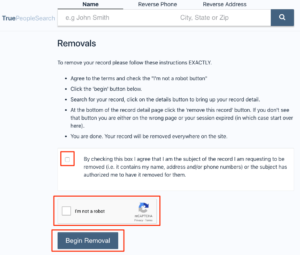This image is a screenshot of a webpage, taken either from a phone or a computer. The screenshot is square-shaped and features small, hard-to-read text. At the top of the screenshot, there is a grey header with three tabs: "Name" (which is highlighted with a black underline), "Reverse Phone," and "Reverse Address."

Below the header, on the left side, is a logo for "True People Search," with "True" in a darker font. Adjacent to the logo is a white search box containing the placeholder text "Example: John Smith," followed by fields for "City, State or ZIP" and a search button.

Beneath the search box, there is a section labeled "Removals" in black text. This section includes a series of five bullet points that seem to provide step-by-step instructions, although the text is too small to read clearly.

Further down, there is a long, rectangular white box with black text, likely containing terms of agreement, and an unchecked white checkbox with an orange highlight around it. Adjacent to this is a CAPTCHA box labeled "I am not a robot," which also contains an unchecked box. Below the CAPTCHA is a green button with white text saying "Begin Removal," which is also surrounded by an orange highlight.

The image appears to show the steps and elements needed for navigating the website, specifically focusing on the process for removing personal information.